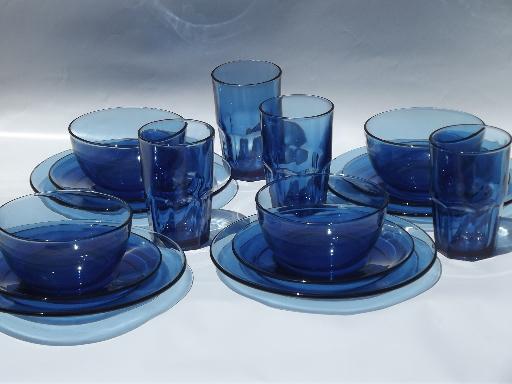The image displays a meticulously arranged set of semi-transparent cobalt blue tableware against a crisp white background. Each set includes a flat plate at the base, topped by a curved plate, and finally a large deep bowl that appears more intense in blue where the pieces intersect. The arrangement features four main sets: one on the bottom left, slightly above the corner; another directly to its top right; a third on the bottom right; and the last set on the top right. Positioned between these sets are four taller glasses, two situated between the sets, one outside the top two, and another to the far right. The interplay of light and shadow casts soft baby blue reflections on the white surface below, enhancing the elegant display.